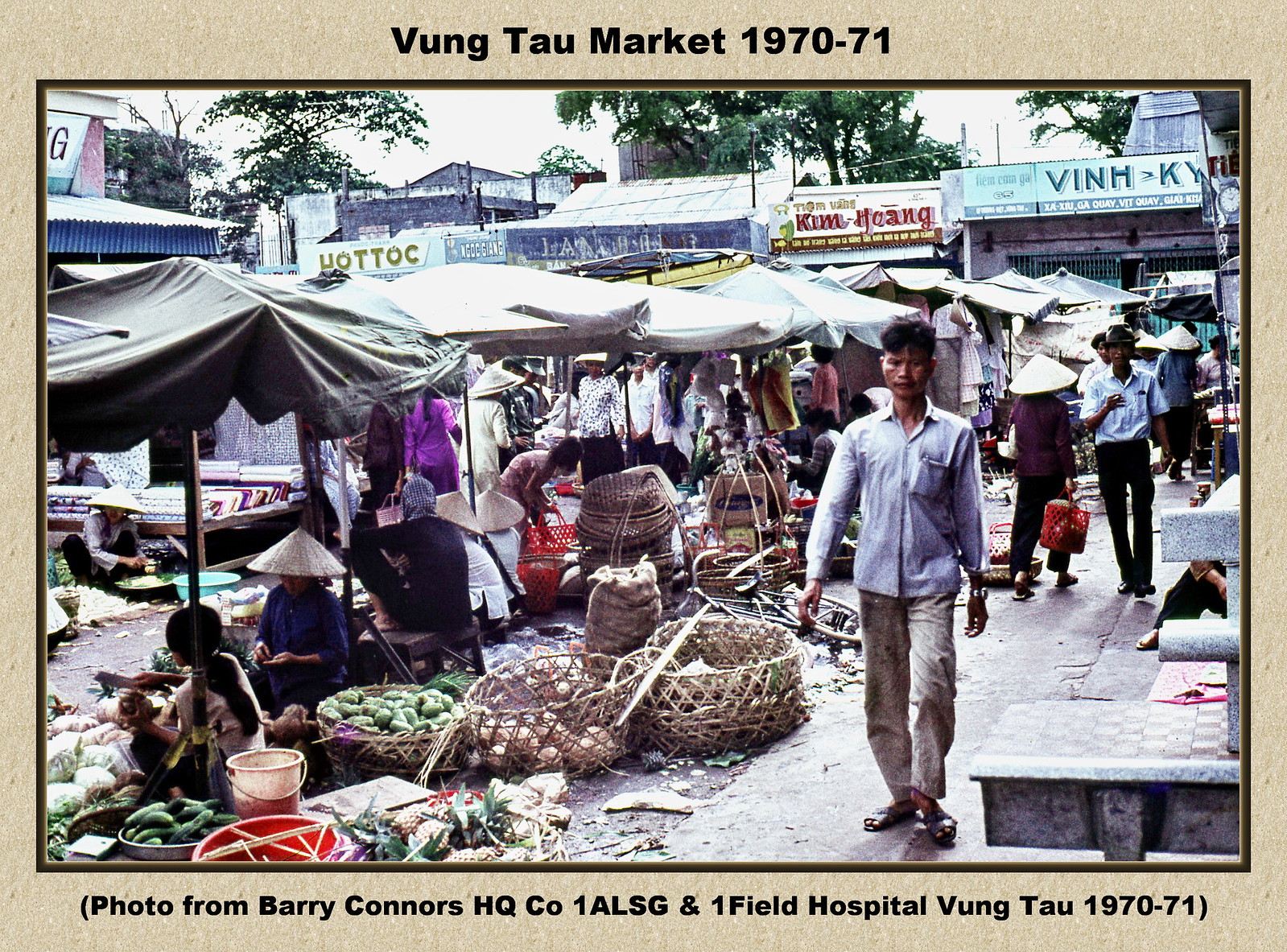This wide rectangular digitally framed photograph depicts a bustling scene at the Vung Tau Market in Vietnam between 1970 and 1971. The frame itself is textured and beige with a burnt brownish-green inner border. Bold black text at the top reads "Vung Tau Market, 1970 to 71," and the bottom caption in parentheses states, "(Photo from Barry Connors HQ, Co. 1ALSG and One Field Hospital, Vung Tau, 1970 to 71)."

The photograph captures a vibrant outdoor market with numerous tents, which start from the middle left and extend to the image's right edge, sheltering women and children donning cone-shaped hats. People bustle around, including a man in the foreground in a white shirt and light pants, walking towards the camera. The background reveals a row of storefronts with Vietnamese signage, while trees can be seen further back. The market scene is rich with color, including shades of tan, black, brown, purple, light blue, yellow, red, maroon, green, and gray, illustrating the diversity of goods and garments in this lively setting.